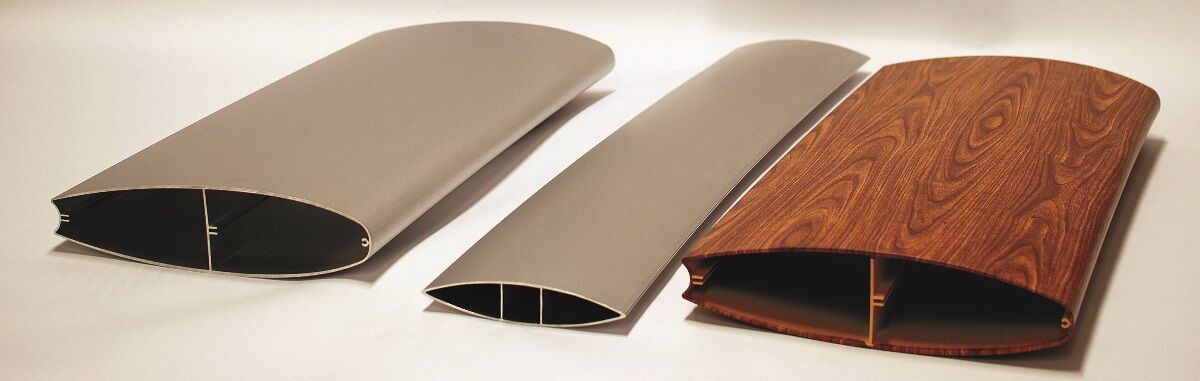The photograph features three distinct cylindrical objects, slightly flattened, positioned against a white and grey gradient background. Each object is hollow with an opening facing the viewer. The leftmost object, the widest of the three, is a matte grey cylinder with a surfboard-like shape. It has a white partition centrally located inside, visible through the opening angled slightly to the left. The central object is similarly shaped but narrower and smaller, resembling an almond with two white partitions forming a square within the center of the almond-shaped opening. The rightmost object, identical in size to the left one, boasts a marbled red wooden texture with visible woody swirl designs. Its flat tube-like structure also has an internal vertical wooden strip supporting it. Each object maintains a modern and sleek appearance, with the grey ones exhibiting a metallic texture, contrasting the natural aesthetic of the wooden one.